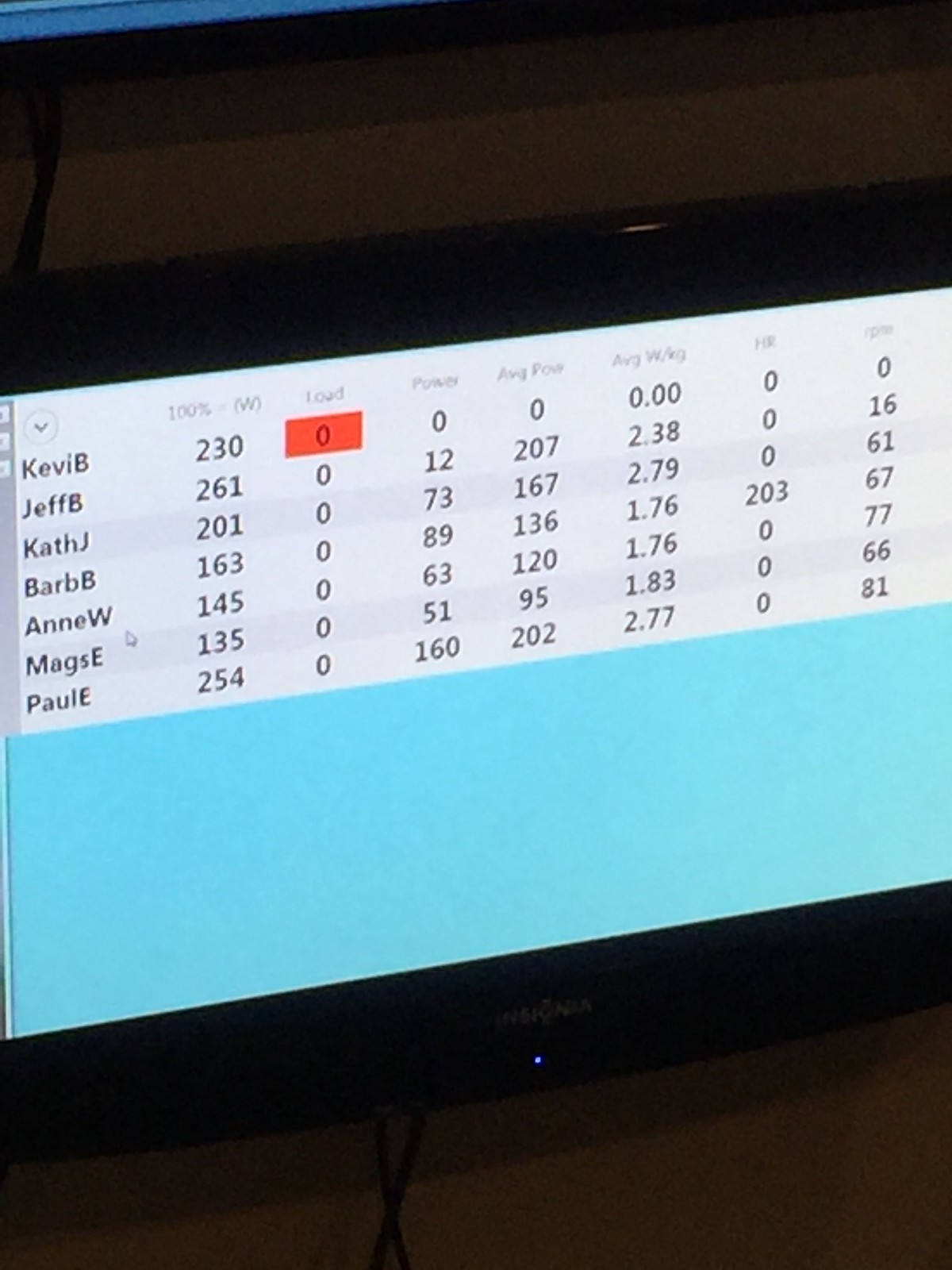The image depicts a photograph of an Insignia-branded television screen displaying a detailed statistics board. The screen is divided into two main areas: the top half features a white background with rows of names and numbers, while the bottom half has a light blue or teal hue. The black bezel at the bottom of the TV prominently displays the "Insignia" logo.

On the left column, the names listed are Kevin B, Jeff B, Cath J, Barb B, Ann W, Mags E, and Paul E. To the right of the names, there are seven columns displaying various numbers. The first column of numbers states: 230, 261, 201, 163, 145, 135, and 254. The subsequent columns feature a mixture of zeros and other numerical values, with some entries highlighted in an orange box. 

Text above these columns, which should clarify the meaning of the data, is blurred and illegible. However, there are hints that the stats might include metrics such as "average weight per kilogram (W/KG)," "HR," and "points," suggesting the data could be related to fitness or athletic performance like CrossFit or weightlifting. The environment around the TV is dimly lit, emphasizing the glowing screen filled with detailed, albeit somewhat cryptic, statistical information.